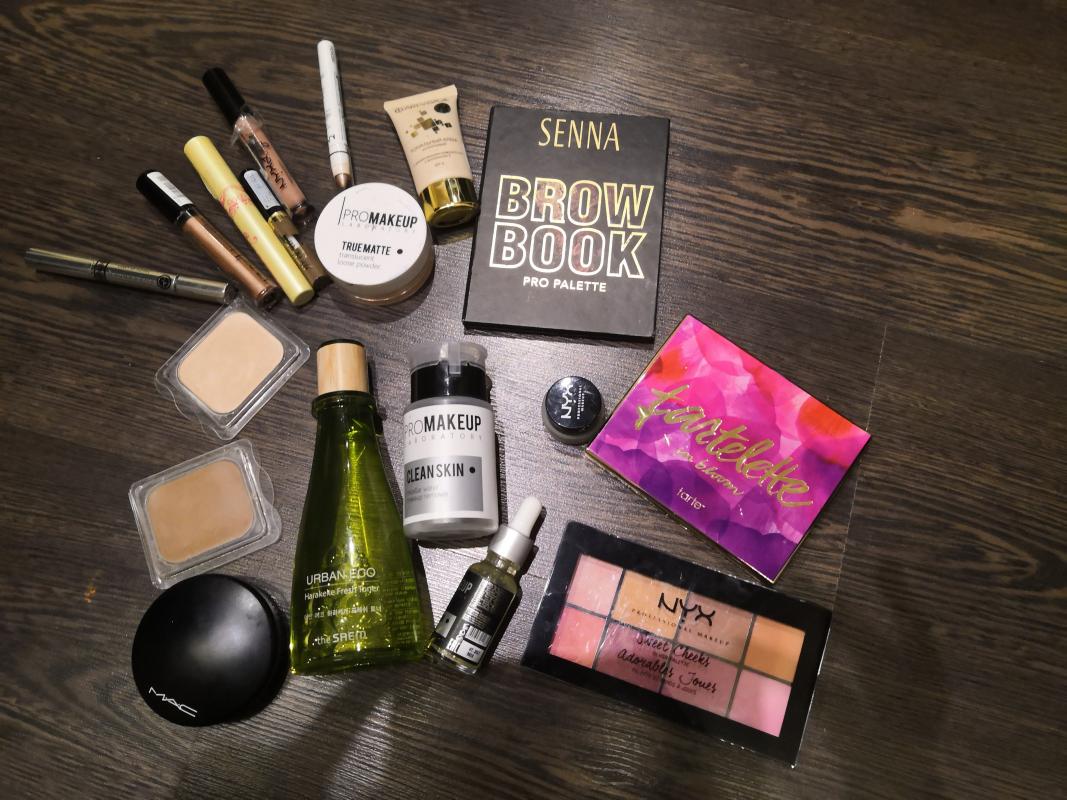The image depicts a wooden table, albeit likely an imitation given the visible seam running down the middle. The table appears cluttered with various makeup items and tools. Among the items are makeup debris scattered around. Notably, there is a small plastic jar labeled "Clean Skin Pro Makeup," featuring black accents around its brim. Another prominent item is a stylish emerald green bottle with a wooden cap, partially labeled "Urbango" or "Urban...". At the top of the image lies a product resembling a book, labeled "Sina Brown Book Pro Palette," accompanied by additional makeup items such as eyeliner and lipstick. Adjacent to these is a colorful card, predominantly red, pink, and purple, which appears to be labeled "Fartelit" or something similar.